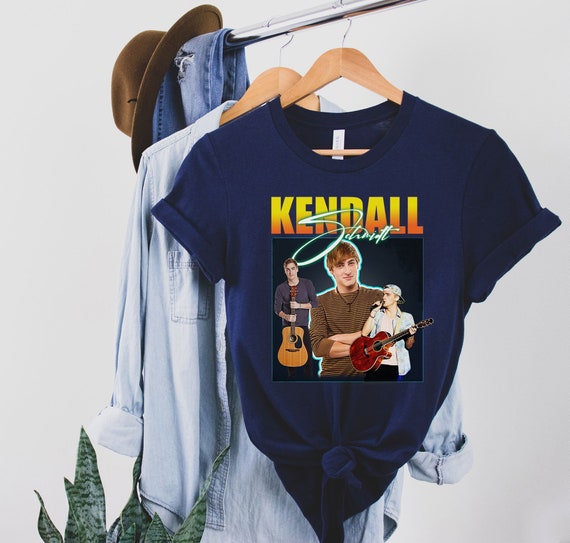This color photograph displays an arrangement of clothing hanging from a horizontal metal rod, reminiscent of a closet setting. Dominating the scene is a blue t-shirt on a wooden hanger. The shirt features the name "KENDALL" in bold yellow capital letters over a cursive "Schmidt." It showcases three images of the pop musician Kendall Schmidt, with the central image flanked by two where he holds acoustic guitars—one brown and the other a reddish-brown. Behind the t-shirt, a denim button-down shirt with rolled cuffs hangs, accompanied by a pair of blue jeans. A brown hat reminiscent of Indiana Jones's style is perched on the bar’s corner. A green plant adds a touch of nature in the bottom left corner against a light gray wall backdrop.